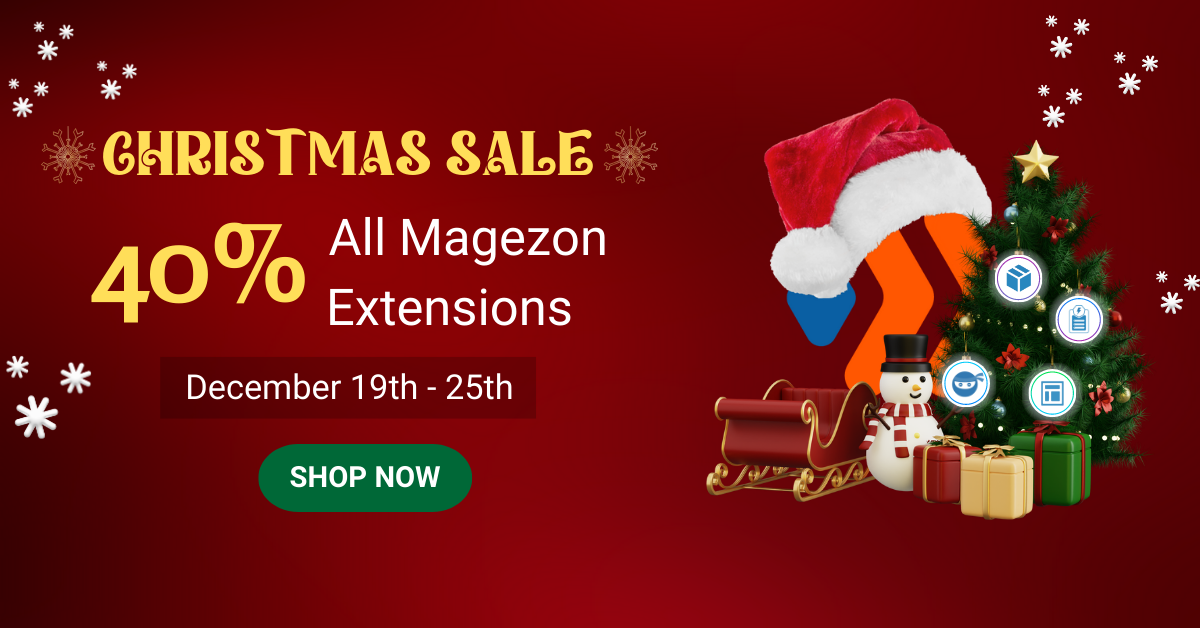The image appears to be a promotional graphic taken from a website. The background is a festive red adorned with white stars in the corners. Prominently, it announces a "Christmas Sale" with the offer of "40% off All Magazine Extensions." Below this, the sale duration is specified as from December 19th through the 25th. There is a "Shop Now" button, likely designed to redirect viewers to the shopping page. In the lower section, there is a company logo featuring blue and green colors, adorned with a Santa Claus hat to match the holiday theme. Accompanying the logo are several Christmas-themed elements, including a decorated Christmas tree topped with a gold star and embellished with various ornaments, three wrapped presents, a sleigh, and a cheerful snowman.